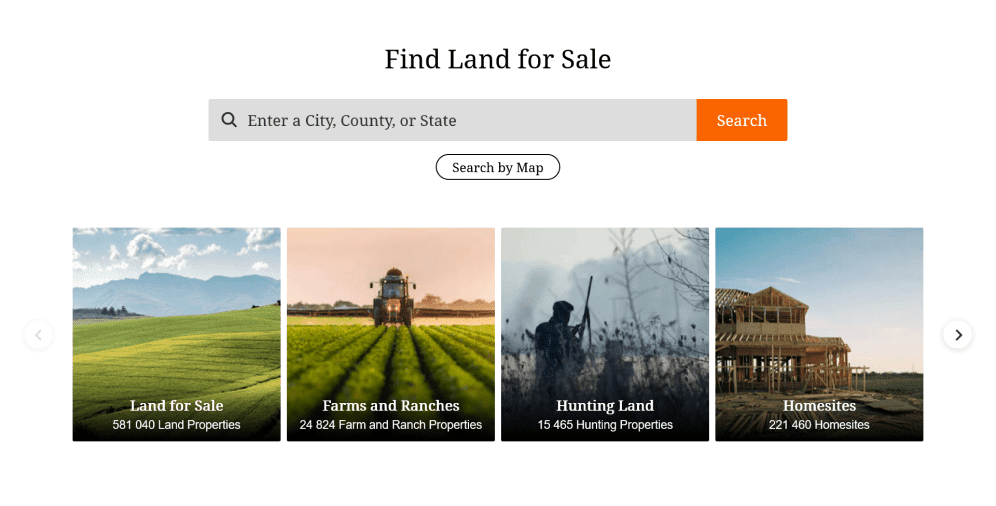In the image, we see a well-organized website interface dedicated to searching for land for sale. At the top of the page, a bold black headline reads "Find Land for Sale," serving as an introductory prompt for users. Directly beneath this headline, a search bar contains the text "Enter a city, county, or state" within a subtle gray box, complemented by a magnifying glass icon on the left. To the right of the search box, a prominent orange button labeled "Search" invites user interaction.

Further down, a "Search by Map" bar offers an alternative search method. Below this, the interface is divided into four distinct squares, each representing a different land category with a visual icon and the number of available properties.

1. The first square, titled "Land for Sale," includes a detailed count of 581,040 land properties.
2. The second square, labeled "Farm and Ranches," features an image depicting a farm with a tractor, indicating 24,824 available farm and ranch properties.
3. The third square, "Hunting Land," showcases an image of a person holding a rifle, ready for hunting, and lists 15,455 hunting properties.
4. The final square, "Home Sites," contains an image of a wooden house structure under construction and mentions there are 221,460 available home sites.

Each category square provides a specialized area of interest, allowing users to find specific types of land that suit their needs.